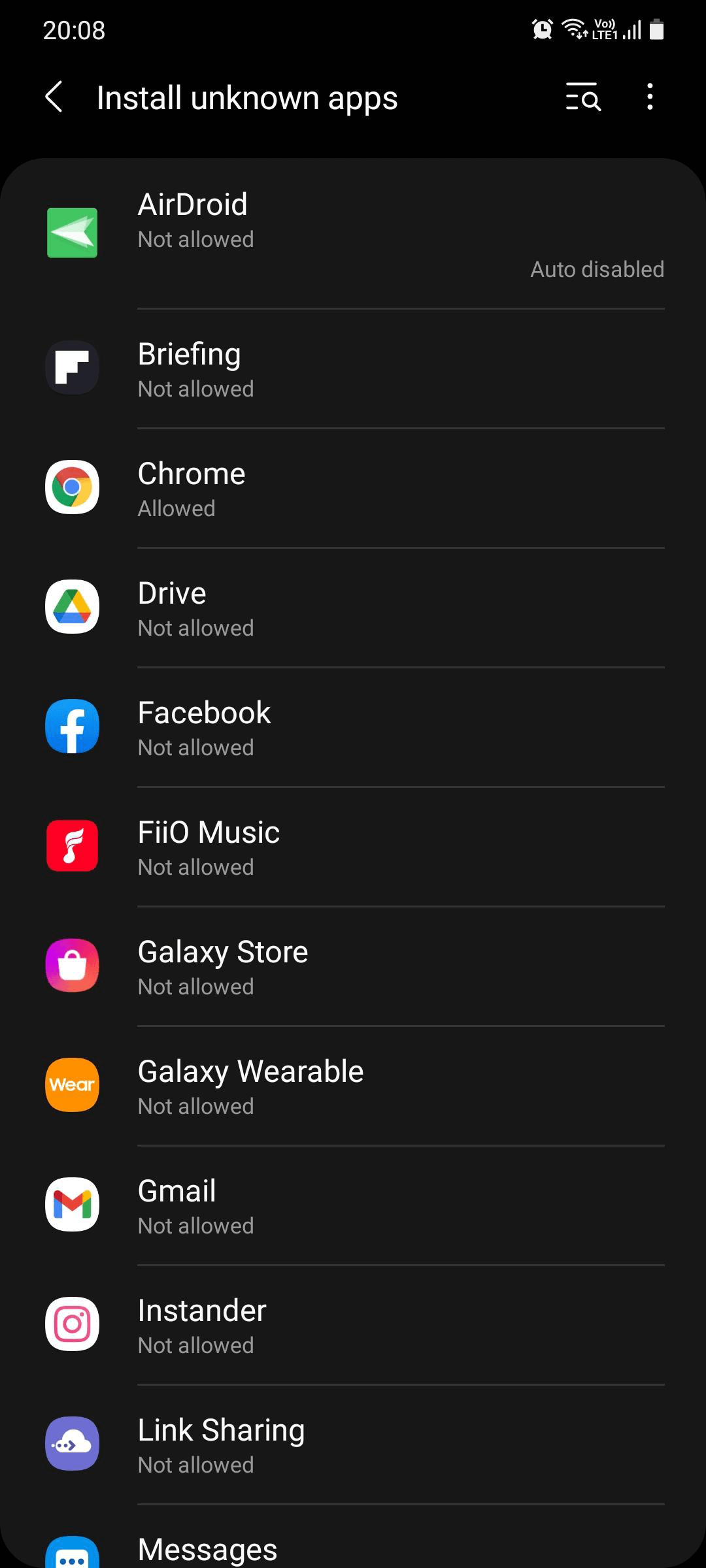The caption is:

"In a screenshot of an iPhone's settings menu, the device is shown in Dark Mode under the 'Install Unknown Apps' section. The menu lists various apps with their respective icons, including AirDroid, Briefing, Chrome, Drive, Facebook, FiiO Music, Galaxy Store, Galaxy Wearable, Gmail, Instander, and Link Sharing Messages. Each app has a status indicator next to it, with most marked as 'Not Allowed' for installing unknown apps. The exception is Chrome, which is indicated as 'Allowed.' This suggests that only the Chrome browser is permitted to install apps from unknown sources, which may refer to apps not officially recognized or approved by Apple."